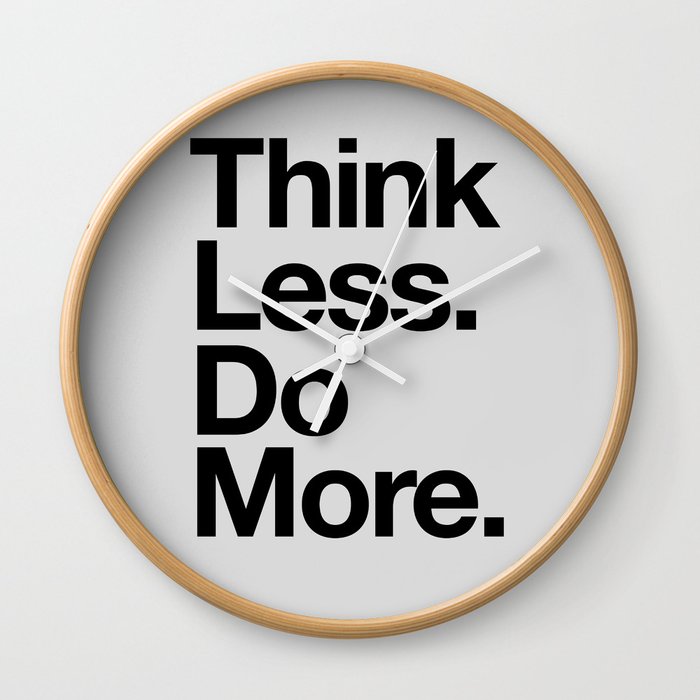The photograph features a modern, thin wooden clock with a brown bamboo-like outline, set against a stark white background. The clock, devoid of any numbers, prominently displays a motivational phrase in large, bold black letters: "Think less. Do more." Each word is positioned on a separate line, with periods following "less" and "more." The clock's hands, including the hour, minute, and second hands, are a bright stark white, subtly contrasting yet not detracting from the powerful message. Slight shadowing from the clock's edges can be discerned, adding depth to its minimalist design. This image emphasizes the clear, motivating message as its focal point, compelling viewers to ponder its meaning.